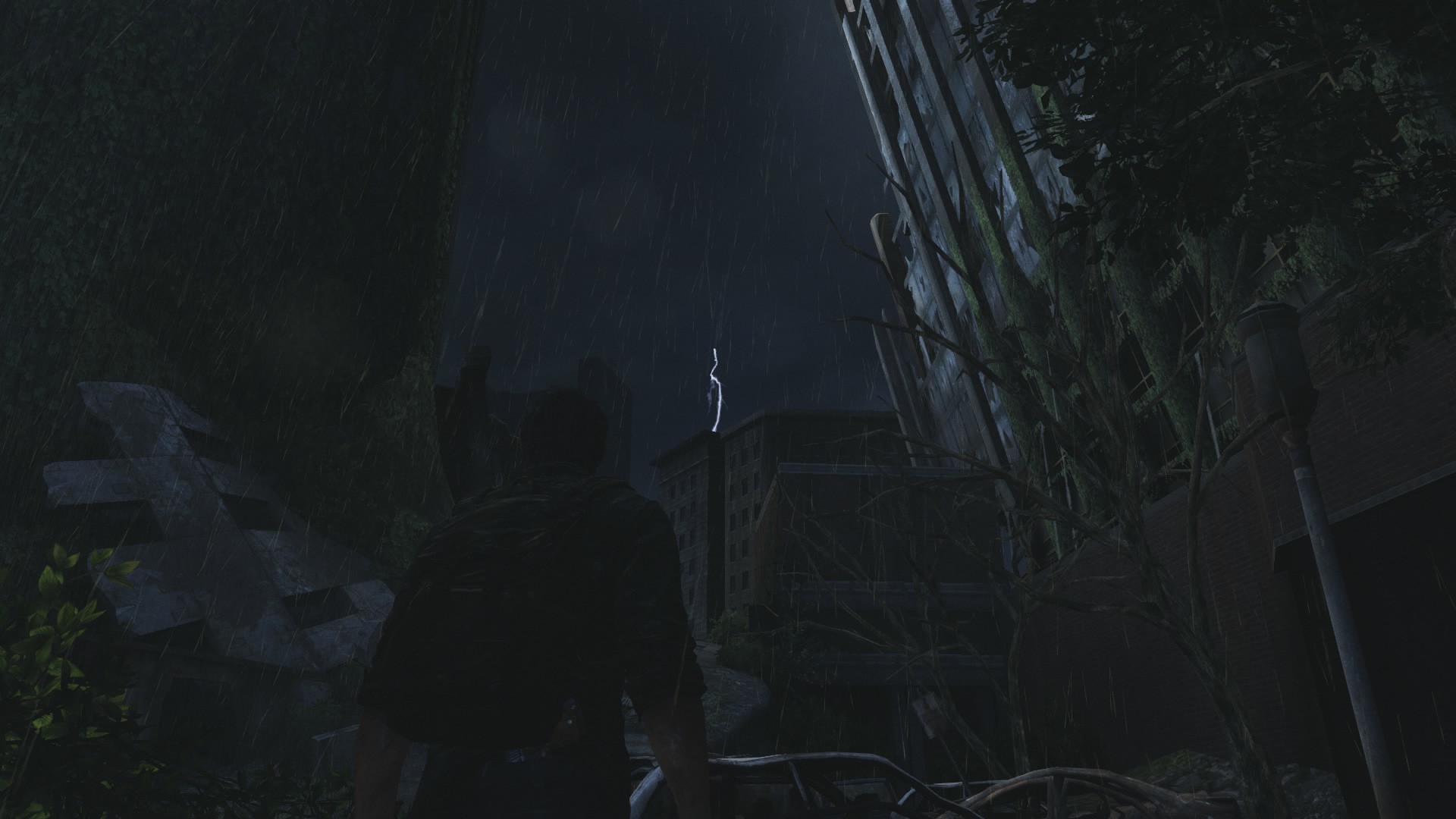In a nighttime setting, a man stands with his back toward us near the bottom left third of the image. To the left of him, there is some vegetation. Nearby, a slanted structure made of concrete blocks seems to serve as a retaining wall for the landscaping. Further to the right, a tall building slopes outward to the left, while in the background, a shorter concrete building and possibly other structures are visible. At the bottom of the image, the tops of three cars can be seen.